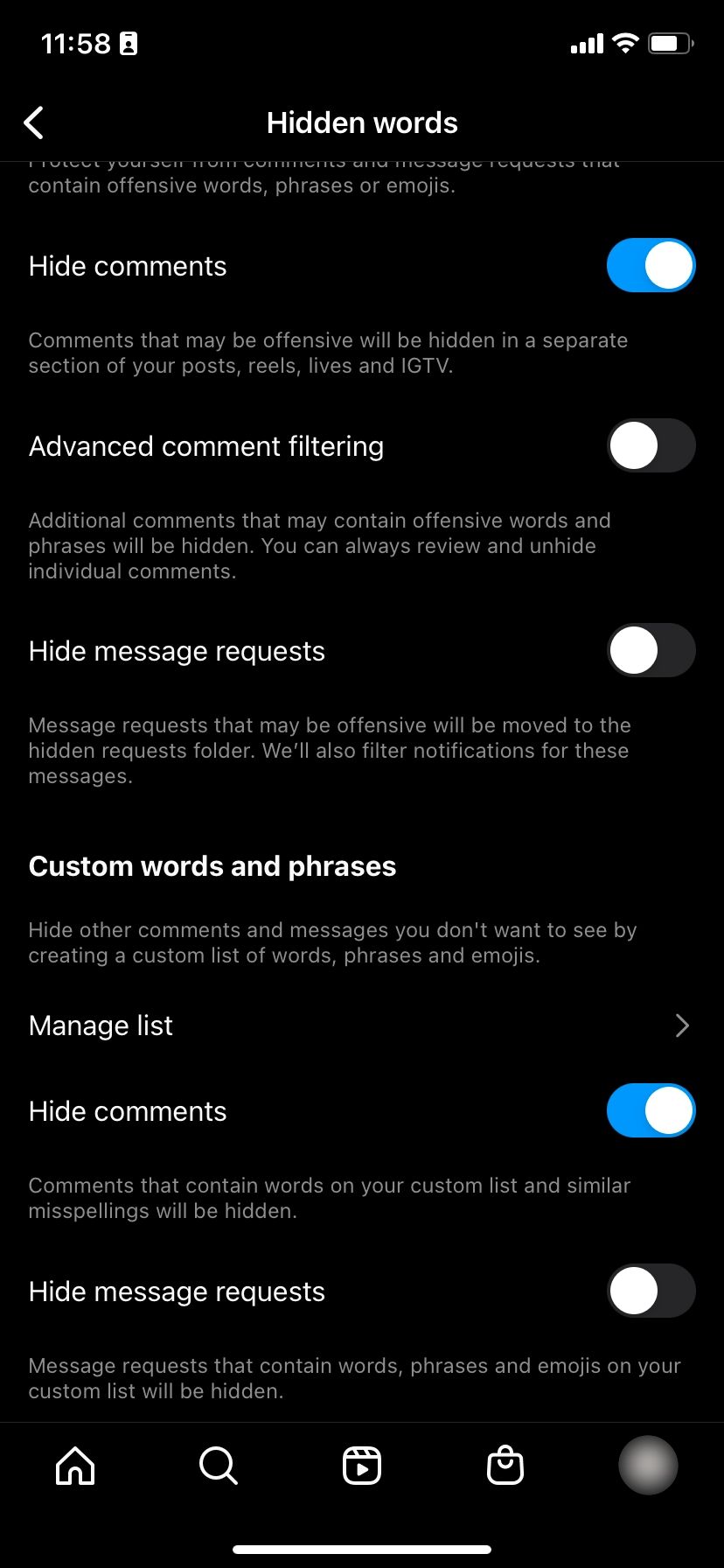Screenshot of a phone displaying the Instagram app, captured at 11:58 AM in portrait mode. The phone layout features a black background with all text appearing in shades of gray or white. The device is connected to Wi-Fi and has a nearly full battery.

At the top of the screen, there's a "Back" button, leading to a menu titled "Hidden Words." The primary option here is "Hide comments," which is checked. This setting moves potentially offensive comments into a separate section. The menu mentions that comments may be hidden due to advanced comment filtering being turned off. Additional comments containing specific words or phrases can also be hidden.

The "Hide message requests" option is not enabled. Normally, message requests containing offensive content would be moved to a different folder, with notifications for such messages filtered. There is also a section for "Custom words and phrases," which allows users to hide comments and messages containing predetermined custom words, phrases, or emojis. This section includes an option to manage the custom list.

At the bottom of the screen are navigation tabs including "Home," "Search," "Reels," "Shop," and another icon that is partially obscured but is part of the app's main menu. The screen evidently belongs to someone configuring their Instagram app settings, specifically focusing on managing potentially offensive content.